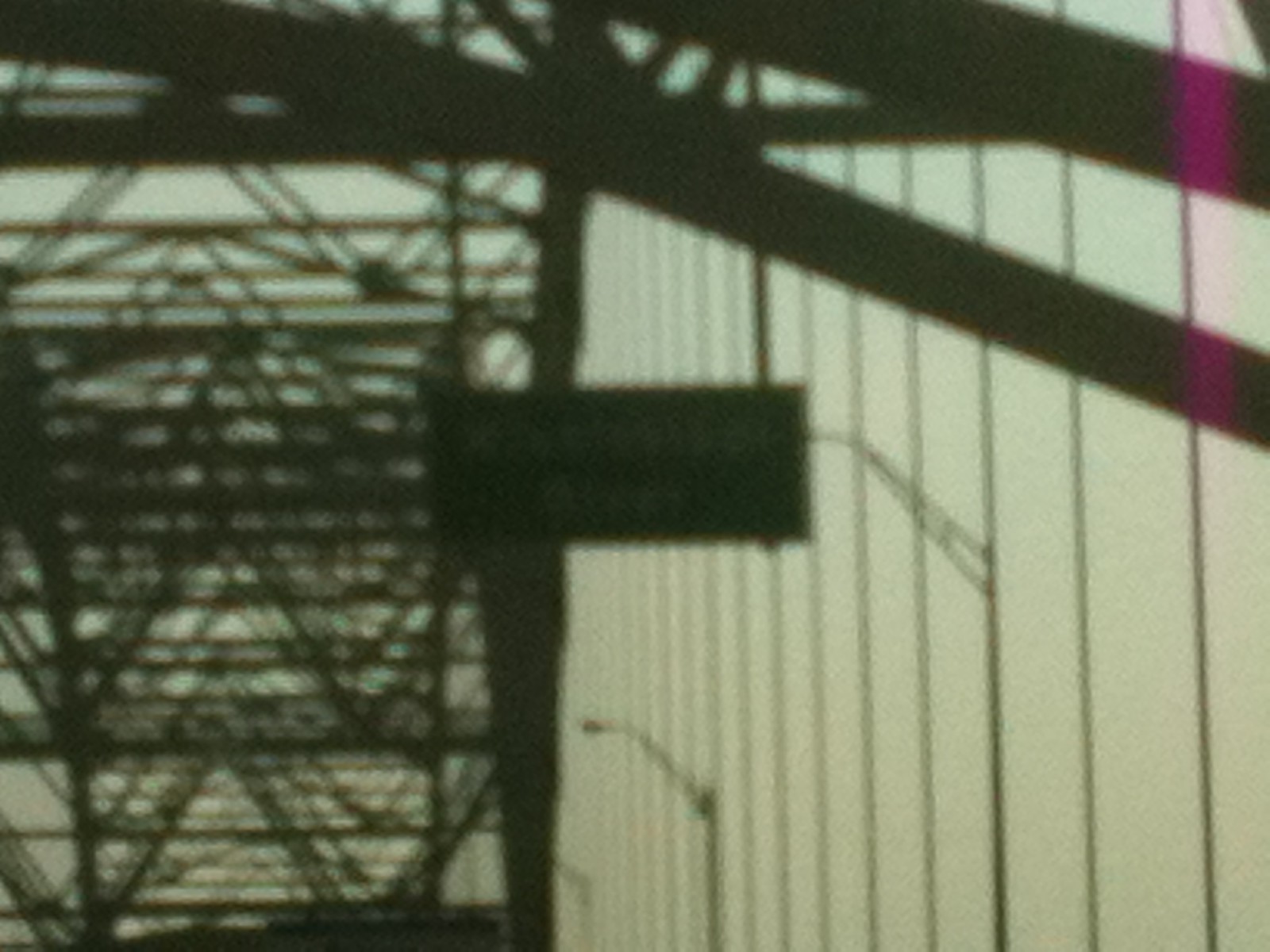A blurry image captures the silhouette of a metal suspension bridge, reminiscent of the Golden Gate Bridge or the Allegheny Bridge in Pittsburgh. The structure, characterized by its metal framework and cables draped to the right, spans over a river, as indicated by a green sign barely visible in the center that reads "something river." The sky in the background is a solid, pale yellow, casting the bridge into deep shadow, making details difficult to discern. Despite the obscurity, the image suggests a viewpoint from beneath the bridge, emphasizing its grand, overhanging presence.